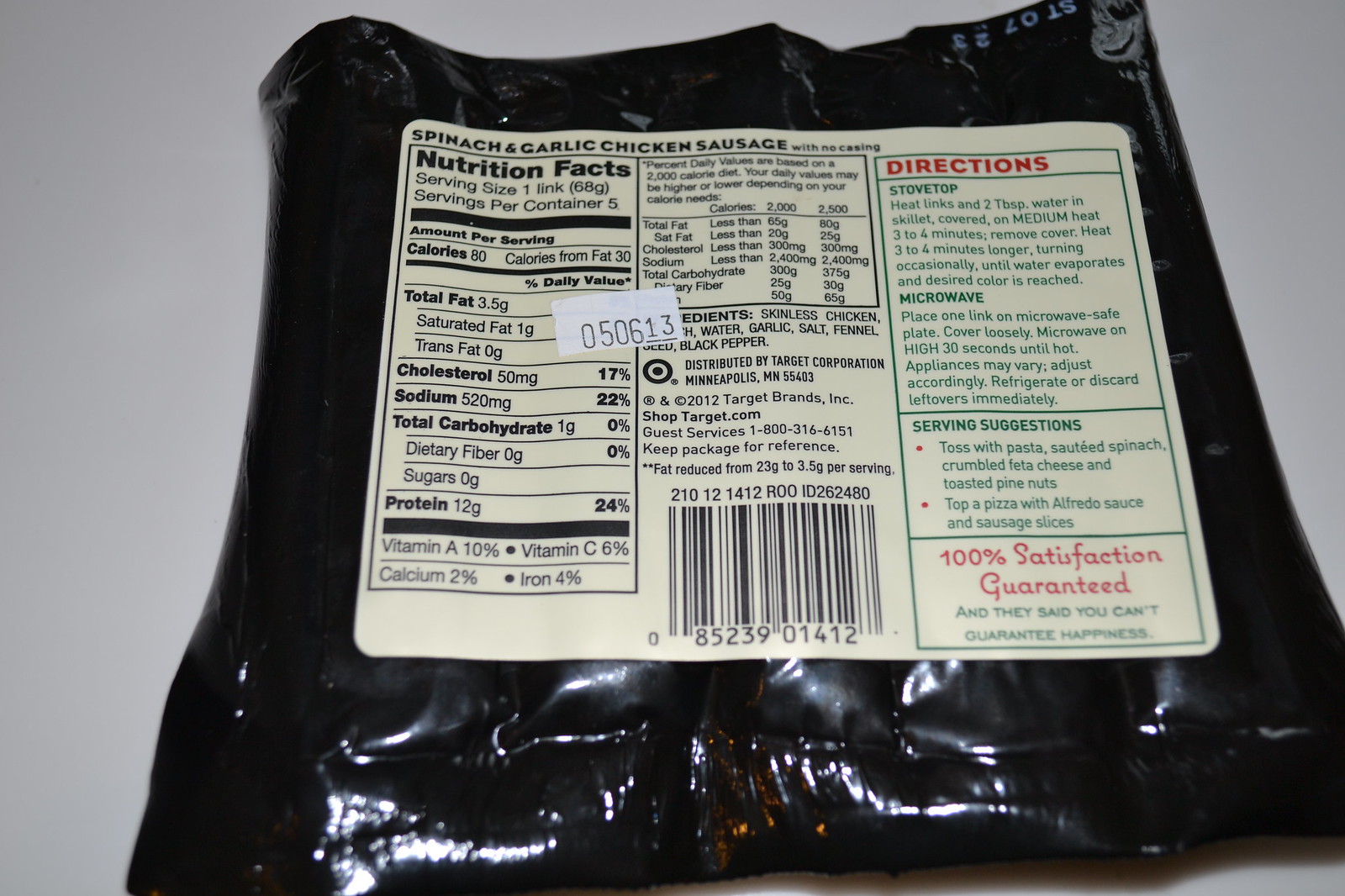This image is a close-up of a package of sausages, captured from the back with a clear view of the label. The background is a subtle light purplish-gray hue, while the package itself is made of black plastic, lying face down on a surface. The label is off-white and provides extensive information about the product. 

At the top of the label, bold text indicates that the product is "Spinach and Garlic Chicken Sausage with No Casing." On the left side, encased within a black border, are the nutrition facts: 80 calories per serving, with a serving size of one link. The label also notes that each serving contains 12 grams of protein, 520 milligrams of sodium, and 3.5 grams of total fat.

The middle section of the label provides daily percentage values based on a 2000-calorie diet. To the right, the word "Directions" is highlighted in red, detailing instructions for both stovetop and microwave preparation. Below these directions are serving suggestions. 

At the bottom of the label, also in red, is a statement: "100% Satisfaction Guaranteed." Below this, in green font, there is a humorous remark: "And they said you can't guarantee happiness."